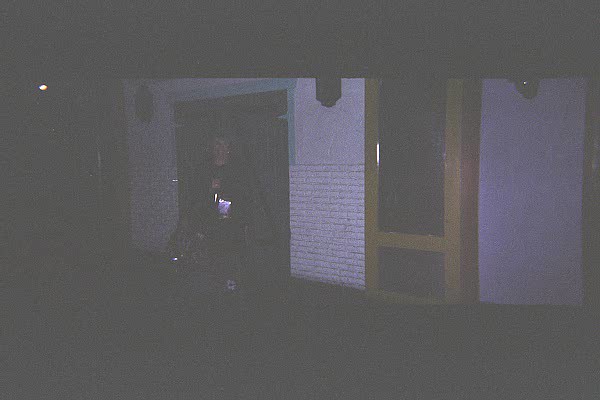The photograph captures a poorly lit nighttime scene, characterized by its grainy and slightly out-of-focus quality, reminiscent of an image taken with an old 1970s or 1980s camera. The setting includes a large double doorway at the center, composed of closed wooden doors and surrounded by a white brick wall. Adjacent to the doorway, light sconces are fixed at the top of the walls, although they are not illuminated. The doorway area could suggest an entrance to a restaurant or similar establishment. 

To the right of the central doorway, there is a dark wooden column with a lighter wood outlining it, which transitions back to more white wall. The entire background scene is very dark, with the upper and lower portions of the image nearly completely black. A faint single light source on the left adds a dim spot of visibility. 

In the foreground, slightly left of center, the indistinct outline of a person dressed in black can be seen walking away from the double doors. The person is holding an indeterminate object that appears white against their dark attire. The overall effect of the photograph is obscure and enigmatic, dominated by shadow and indistinct features, capturing the fleeting moment of someone exiting a dark, atmospheric location.